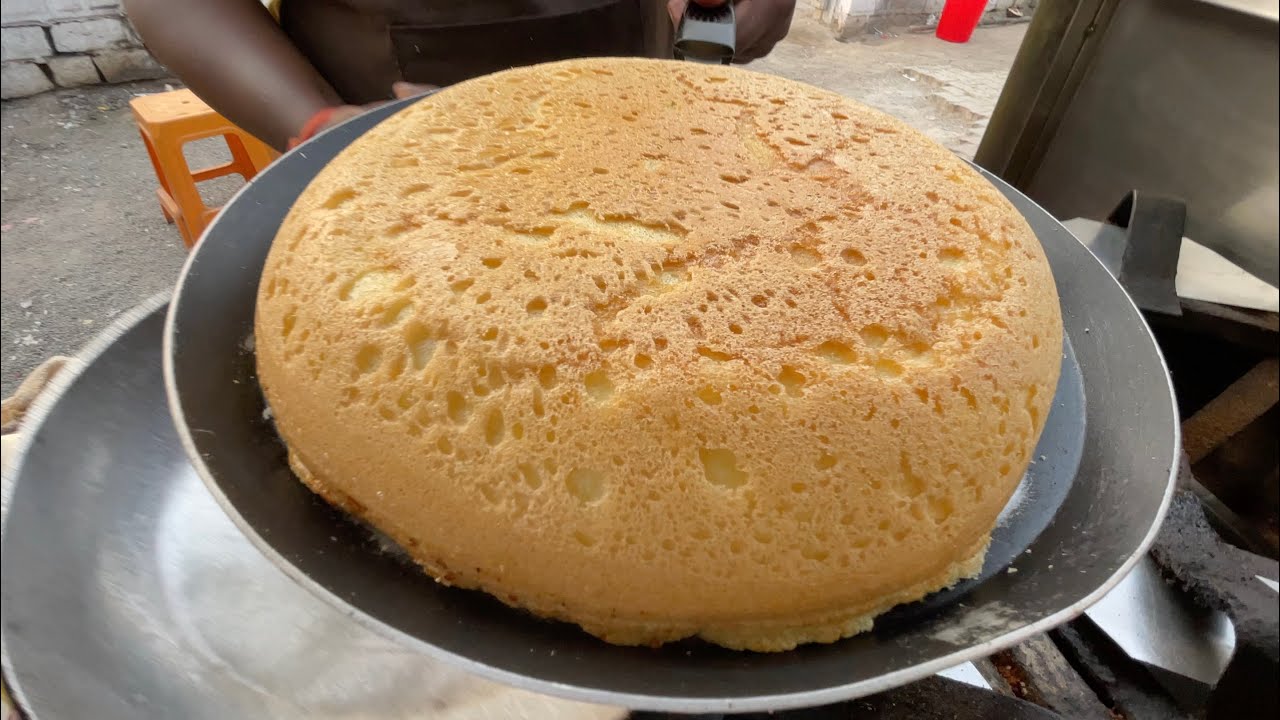In the image, a round, fluffy baked item resembling a sponge cake or a massive pancake rests on a pan, which features black and silver edges and a handle. The cake has a beige, tannish color with visible divots and air pockets, indicating its uneven, textured surface. The bottom appears slightly ripped, suggesting it was just removed from a baking dish. The pan is held by an African-American person's hand, suggesting an outdoor cooking setting. The background reveals a rustic environment with discolored white bricks, an unfinished floor that looks like dirt or concrete, and hints of metal pieces. An orange stool is also visible, adding to the impression of a humble or makeshift kitchen, possibly outside a home or in a poorer dwelling.